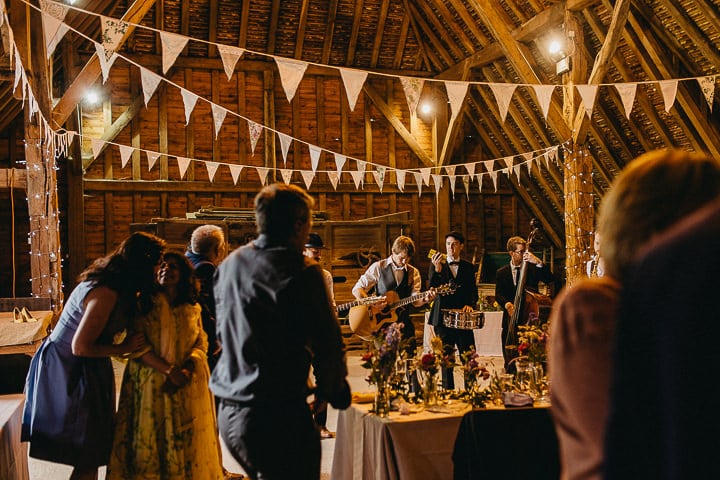This photograph captures a lively and rustic wedding celebration set inside a large wooden barn adorned with wooden beams and lumber. Strung across the room are white triangular flags and fairy lights, adding a festive atmosphere. At the event's center, a band dressed in formal suits is performing; three visible band members are playing instruments, with two in black jackets and one possibly obscured by the audience. A crowd of men and women stands, some sitting, attentively watching the performance. In the foreground, there's a table draped in brown fabric and covered with numerous flower arrangements in glass vases. Two women are seen conversing nearby, adding to the intimate and joyous ambiance of the gathering.